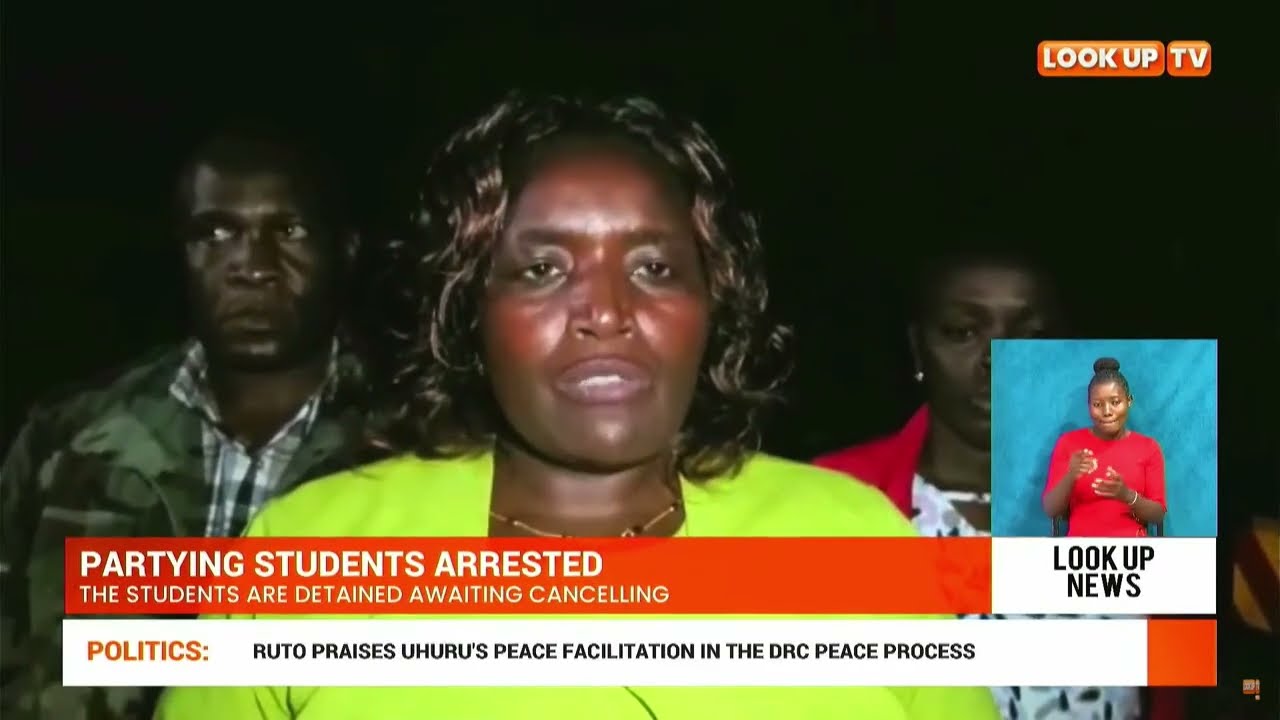The image appears to be a screenshot from a news program. Dominating the center is a distraught-looking dark-skinned woman with dark shoulder-length hair, wearing a bright lime green long-sleeve shirt. Over her right shoulder stands a dark-skinned man dressed in a camo jacket over a white and blue shirt. To her left shoulder is another dark-skinned woman, adorned with a bright earring in her right ear, and dressed in a red dress. The main background behind these three individuals is black. In the lower right corner, there is an inset of a fourth dark-skinned woman with her hair in a bun, wearing a white dress or blouse, who appears to be signing, set against a blue background. The text on the screen includes "Look Up TV" at the top right. Across the bottom, two banners display: the first in black and white lettering on an orange background reads "Partying students arrested. The students are detained awaiting canceling," and the second, in orange lettering on a white background, says "Politics: Ruto praises Uru's peace facilitation in the DRC peace process." The text is colored in black, orange, and white.